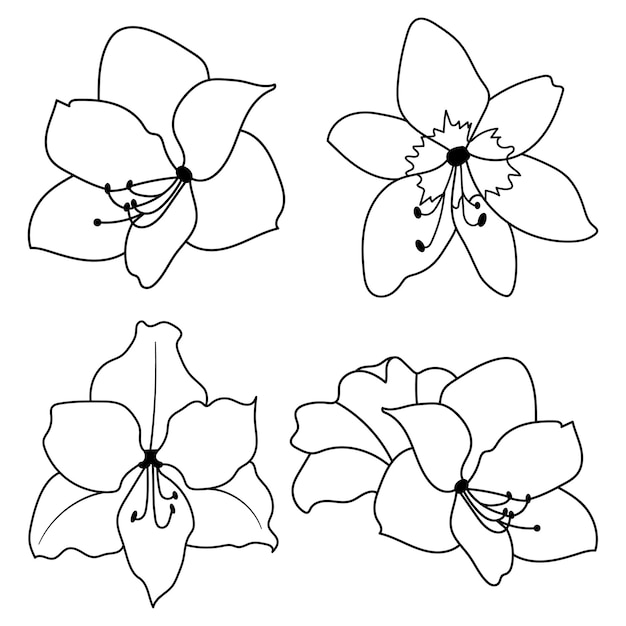This image contains black and white line drawings of four distinct flower blooms, positioned in a grid with two in the top row and two in the bottom row. Each flower is depicted from a different angle with a detailed emphasis on the varying perspectives. The flowers resemble Phalaenopsis orchids, known as the moon or moth orchid, highlighted by its characteristic bright white petals that glow. Each bloom has six visible petals, surrounding an intricate dark center filled with small lines and tiny circles representing the anthers, essential for pollen collection. The flower on the upper right corner reveals traits similar to a dahlia, yet the overlapping descriptions suggest a coherent similarity across all flowers. The line art, while simple, is vividly expressive, giving a sense of liveliness to the blooms.